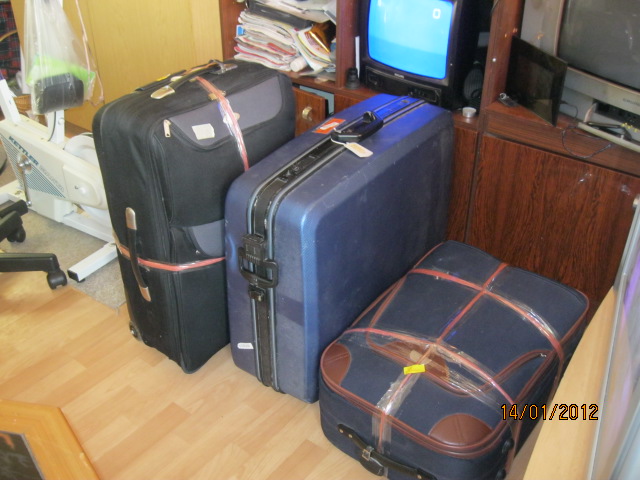The photograph, dated January 14, 2012, captures a room with light-colored, thin plank hardwood flooring and a yellow back wall, possibly inside an office or home. To the right, there's a dark wood TV stand holding two televisions - one operational and another, partially broken with flaps hanging and appearing dirty and inoperative. The stand also has a disarray of papers and books on one of its shelves. To the far left, a white exercise machine, possibly a bike, is visible. An office chair with rolling feet can be seen near the center-left area of the image. In the center lie three suitcases: an upright, tall black suitcase wrapped with red tape; a medium-sized upright blue suitcase with a black stripe and handle, and a small blue suitcase with brown leather edges and red tape, lying on the floor. The date "14-01-12" is visible in small orange text at the bottom right corner of the image.